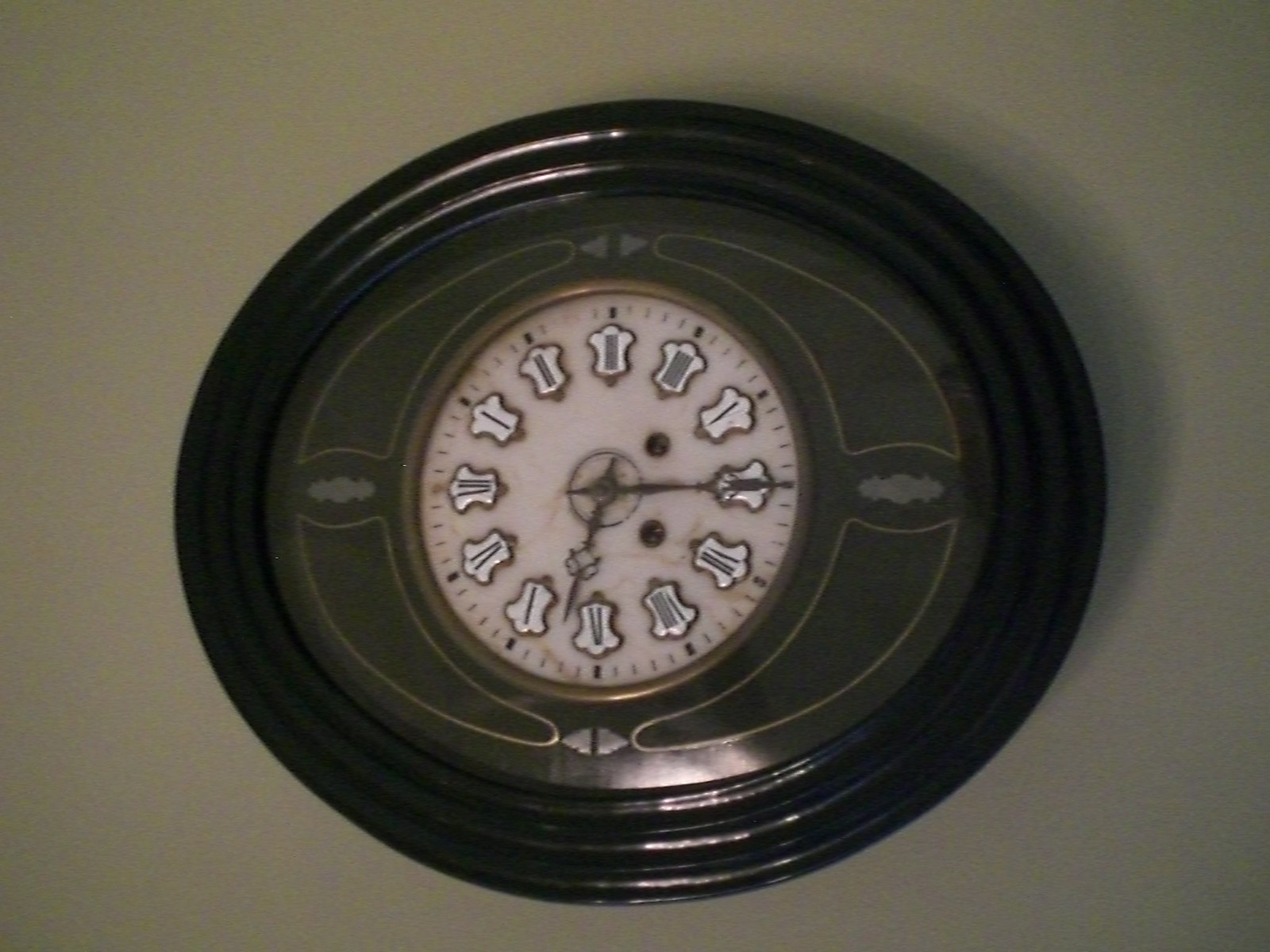This image is a color illustration or photograph, and it depicts a vintage-style wall clock with an intricate design, making it hard to discern if it's a photograph or a digital rendition. The clock features a round, possibly dark brown or black wooden frame with highlighted sections on the top and bottom. The face of the clock is a dark olive green with a marbled light pink or pale pinkish yellow inset where the Roman numerals are displayed, scattered in a flower or tulip shape. 

The clock's hands are ornate, featuring a club-shaped wire design similar to the suit of cards, and there are three small holes on the face, likely for winding and a key. There is an off-white central portion underneath the hands and black detailing on this intricate clock. It is presented against a brown background, casting a shadow in the upper right corner. The clock is currently showing a time of approximately 6:15.